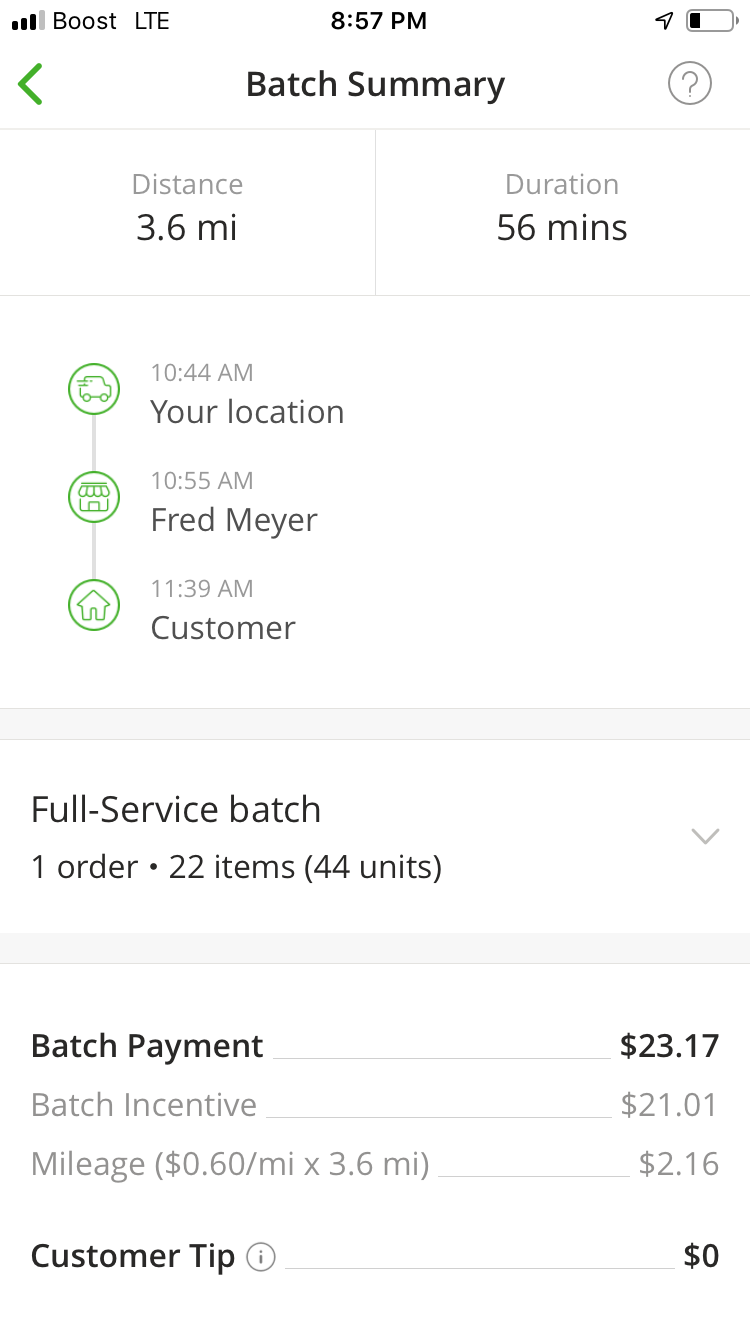Screenshot of a gig application, resembling those used by services like DoorDash, displayed on an iPhone with Boost LTE service at 8:57 p.m. The phone's battery is less than a quarter charged. The image showcases a detailed batch summary from a delivery. The delivery spanned a total distance of 3.6 miles and took 56 minutes to complete. The job started at 10:44 a.m. and involved traveling to Fred Meyer, a grocery store, arriving there at 10:55 a.m. The individual collected 22 items (44 units in total) and completed the delivery by 11:39 a.m. The overall payment for this full-service batch was $23.17, including an incentive of $21.01 and a mileage reimbursement of $0.60 per mile, totaling $2.16 for the 3.6 miles traveled.